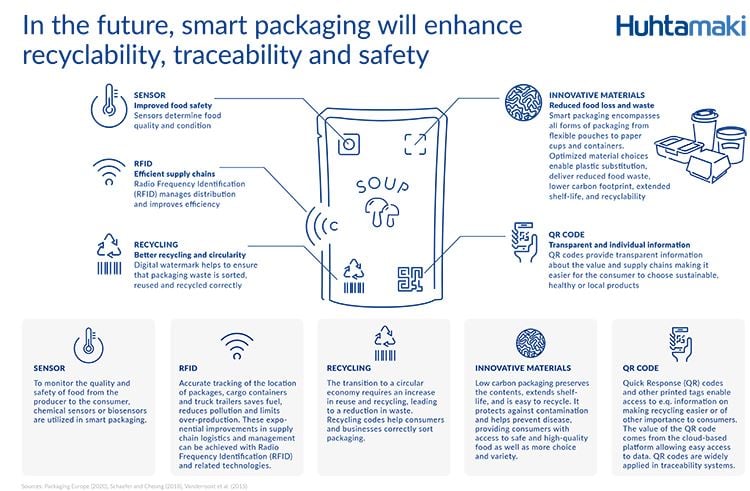The image, seemingly extracted from a brochure, is captioned with the bold blue text, "In the future, smart packaging will enhance recyclability, traceability, and safety." At the top right, the company name "Huhtamaki" is displayed. The central image depicts a soup container with various labels and diagrams radiating outward, each complemented by descriptive paragraphs highlighting key innovations. 

- **Sensor:** Sensors are prominently noted for improving food safety by monitoring food quality and condition. These chemical or biosensors track from producer to consumer, ensuring safety and quality throughout the supply chain.
- **RFID:** Radio Frequency Identification (RFID) is highlighted for its role in efficient supply chain management. This technology aids in accurate tracking of packages, truck trailers, and cargo containers, thus enhancing distribution efficiency, saving fuel, reducing pollution, and limiting overproduction.
- **Recycling:** The diagram emphasizes better recycling and circularity. Smart packaging is designed with digital watermarks to ensure correct sorting, reuse, and recycling. Recycling codes and information support the transition to a more circular economy by guiding consumers and businesses on proper packaging disposal.
- **Innovative Materials:** Smart packaging involves optimized material choices that substitute plastics, reduce food loss and waste, lower carbon footprints, extend shelf life, and are easy to recycle. These materials are designed to protect against contamination, preserve contents, and help prevent disease, thus delivering safe, high-quality food with more choice and variety.
- **QR Code:** QR codes provide transparent individual information about the value and supply chains. These quick response codes facilitate easy access to data, making recycling easier and aiding consumers in making sustainable, healthy, or local product choices. This access is made possible through a cloud-based platform and is an integral part of traceability systems.

Each aspect of the packaging from sensors to QR codes is designed to improve the overall sustainability, efficiency, and safety of food packaging, reinforcing Huhtamaki's vision for the future.